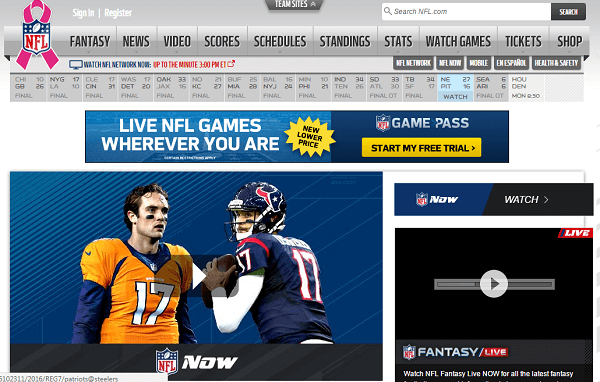This image is a screenshot from an NFL league website, showcasing a typical user interface. At the top right corner, there's a sign-in and login bar for users to access their accounts easily. Just below it, users are presented with various subheadings, including Fantasy, News, Videos, Scores, Schedules, Standings, Stats, Watch Games, Tickets, and the Shop for quick navigation to different sections of the site.

Further down, the page displays a comprehensive list of scores from various NFL leagues, detailing the final scores for each team. There's also a prominent blue-colored button inviting users to watch an NFL game live, emphasizing the availability of live streaming options. Below this feature, there's an option to watch an advertisement prior to accessing the live game stream.

Additionally, the page includes several advertisements promoting a free trial offer for a game pass, allowing users to watch NFL games without a subscription initially. One of the central visuals on the page is an image of an NFL player wearing an orange jersey with the number 17, standing opposite another player in a blue jersey, also number 17, both donned in full gear and helmets. This image likely highlights key players or an upcoming game, adding a dynamic element to the webpage.